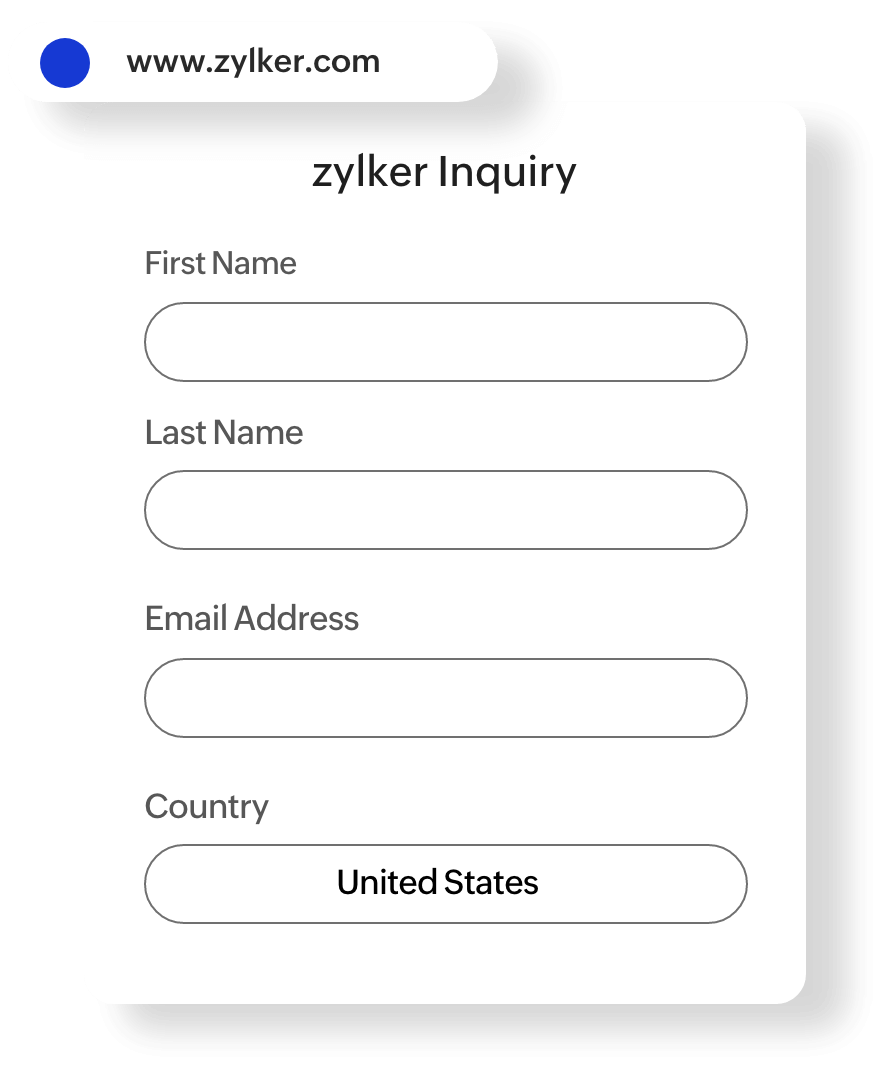The image depicts a webpage on the site www.zykler.com. In the upper left corner, there is a distinctive blue dot representing the website's logo. To its immediate right, the website address is clearly displayed. Slightly below this, there is a subtle shadow effect. The main focus of the image is a form titled "Zylker Inquiry" in bold black letters. The form contains several fields for user input: "First Name," "Last Name," "Email Address," and "Country." The "Country" field is already filled out with "United States," whereas the other fields remain empty. Each input field has an accompanying bubble for users to enter the requested information. The form itself is neatly enclosed in a rectangular shape, whose size is appropriate for its intended purpose.